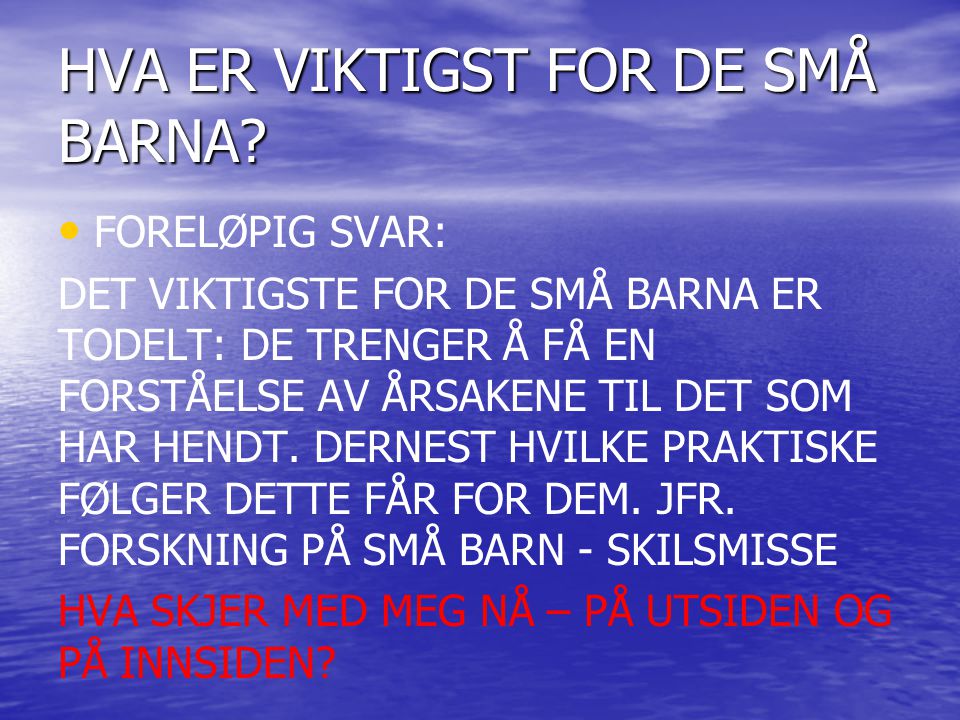The image depicts a bright blue ocean with a clear sky adorned with wispy white clouds. Overlaid onto this serene background is a text in a foreign language that appears Scandinavian. The upper portion of the image features two lines of text in white block letters with black outlines, reading "HVA ER Vektigst for De Sma Barna." Below this, there are six lines of white text without black outlines. The bottom section of the image contains two lines of bright red text, ending with a question mark: "HVR Sker Med Magna Par Utsidin Og Par Insidin?" Additionally, a yellow bullet point is present near the headline, emphasizing the text.